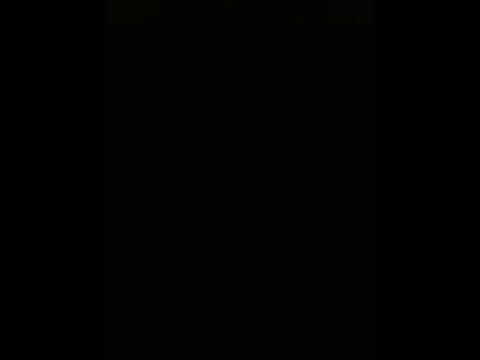The image is a completely opaque, horizontal black rectangle with no indication or thumbnail suggesting otherwise. It spans uniformly from the top to the bottom edge and from the left to the right edge, devoid of any pictures, people, animals, text, or distinguishing features. The entire rectangle is a solid, unbroken black with no shadows, outlines, or variations in color, suggesting it might serve as a background meant for another purpose, though in its current state, it displays nothing but a consistent, uninterrupted blackness.